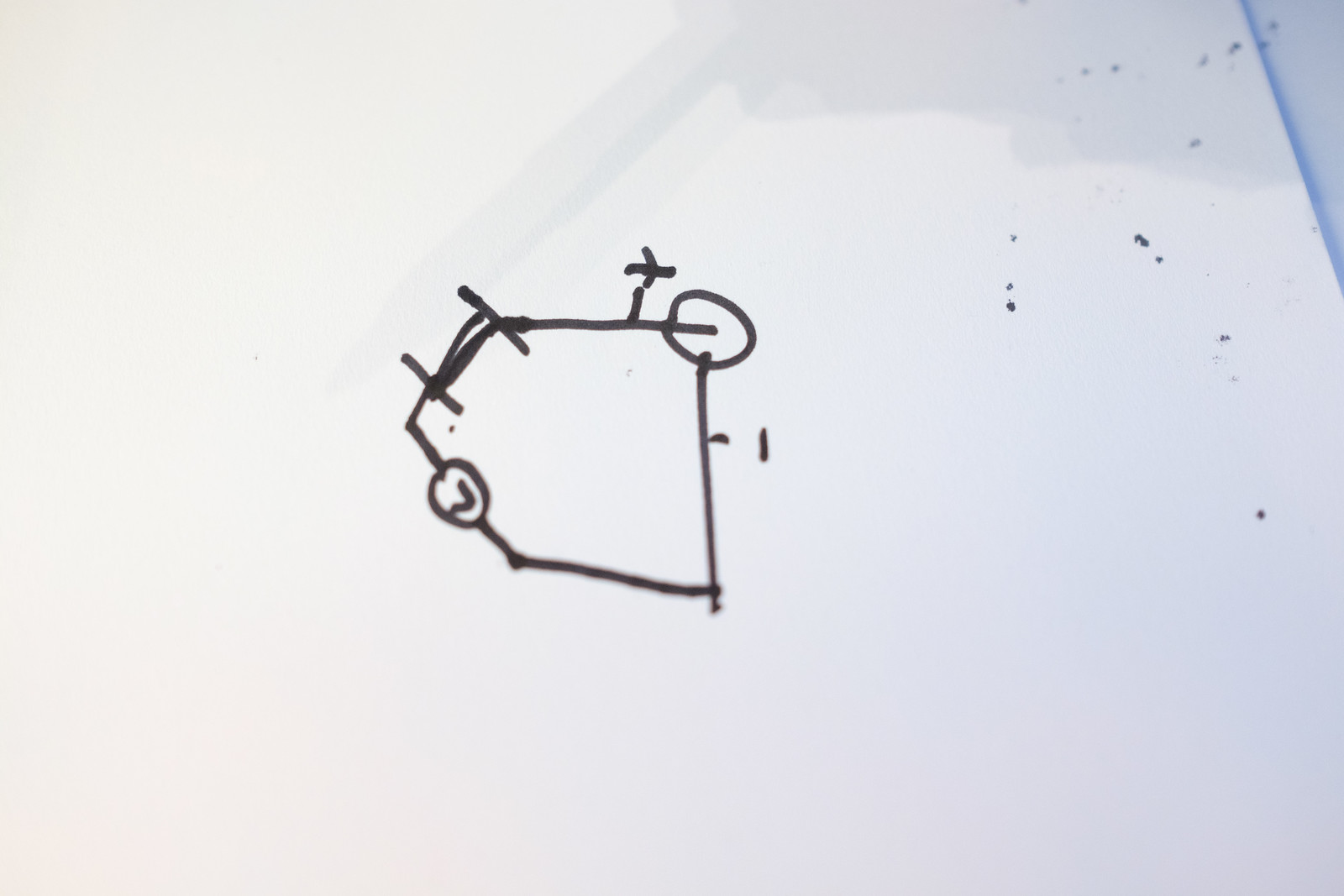This landscape-oriented image features what appears to be a white sheet of paper as its background. In the top right corner, a thin blue triangle is visible, stretching from the upper edge down to the middle of the right side. Scattered along the right side are approximately 8 to 9 small, black dots made with a marker.

Central to the image is a house-shaped object resembling a stout, stocky arrow pointing to the left. On the upper slanted section of this object, there are two straight lines set at a 45-degree diagonal. The top right corner of the house-like shape is encircled. To the immediate left of this circle, there is a straight line dash protruding outwards, accompanied by a small, sideways cross positioned above it in marker. Finally, on the bottom left slanted section of the object, a circle encloses an upside-down V shape.